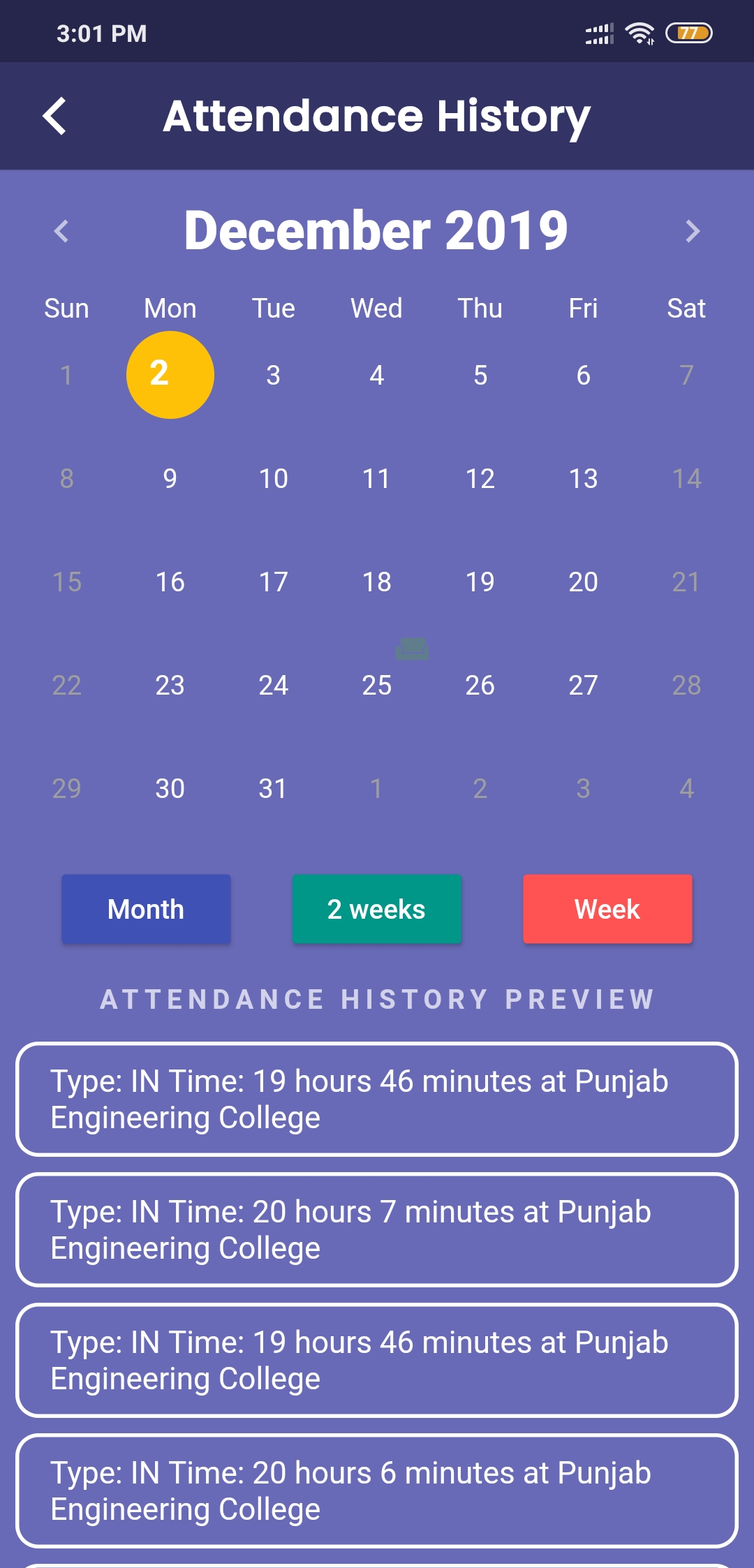The image is a screenshot from a mobile phone displaying an application interface. In the top-right corner of the screen, the battery level is shown at 77% in yellow. The current time, 3:01 PM, is visible in the upper left-hand corner. The main content of the screen centers around "Attendance History," accompanied by a calendar view set to December 2019. A notable detail on the calendar is a yellow circle highlighting December 2nd.

Below the calendar, there are three color-coded boxes aligned horizontally: the first box, labeled "Month," is blue; the second, labeled "Two Weeks," is green; and the third, labeled "Week," is orange. Beneath these options, there is a section titled "Attendance History Preview," which mentions "the time in this Punjab Engineering College."

The overall background of the image is blue, and the main headline at the top is a darker shade of blue, providing a clear distinction between different sections of the interface.